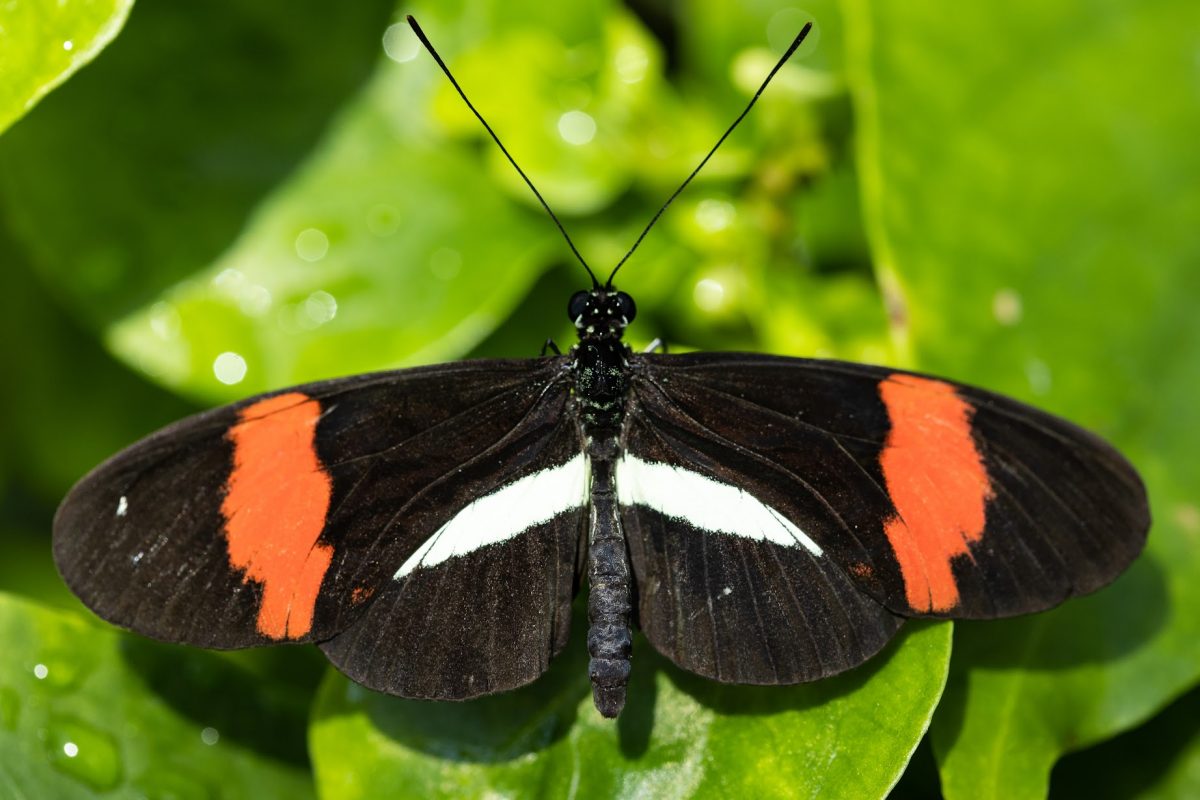The photograph features a close-up, top-down view of a prominently centered black butterfly, slightly below the central horizontal axis. The butterfly's wings are fully outstretched, revealing intricate patterns. Each wing displays a pair of oval-shaped red markings and features a distinct, crescent moon-shaped white area in its midsection. Toward the ends of the wings, near the trailing edges but not at the tips, there are vertical stripes in hues of yellow or orange. The butterfly’s head and body are clearly visible, and from its head extend two long antennae, each curving upwards and slightly outward, almost reaching the top of the frame.

The butterfly is perched on a green leaf, which forms the foreground of the image. Surrounding leaves are visible along the top edges of the photograph, rendered out of focus due to the use of a shallow depth of field, suggesting a humid environment. Dewdrops are scattered across these leaves, and the use of flash creates delicate reflections on both the water droplets and the butterfly’s wings. The overall image has a symmetrical feel, emphasized by the macro lens capturing precise details of the butterfly while the background remains artistically blurred.